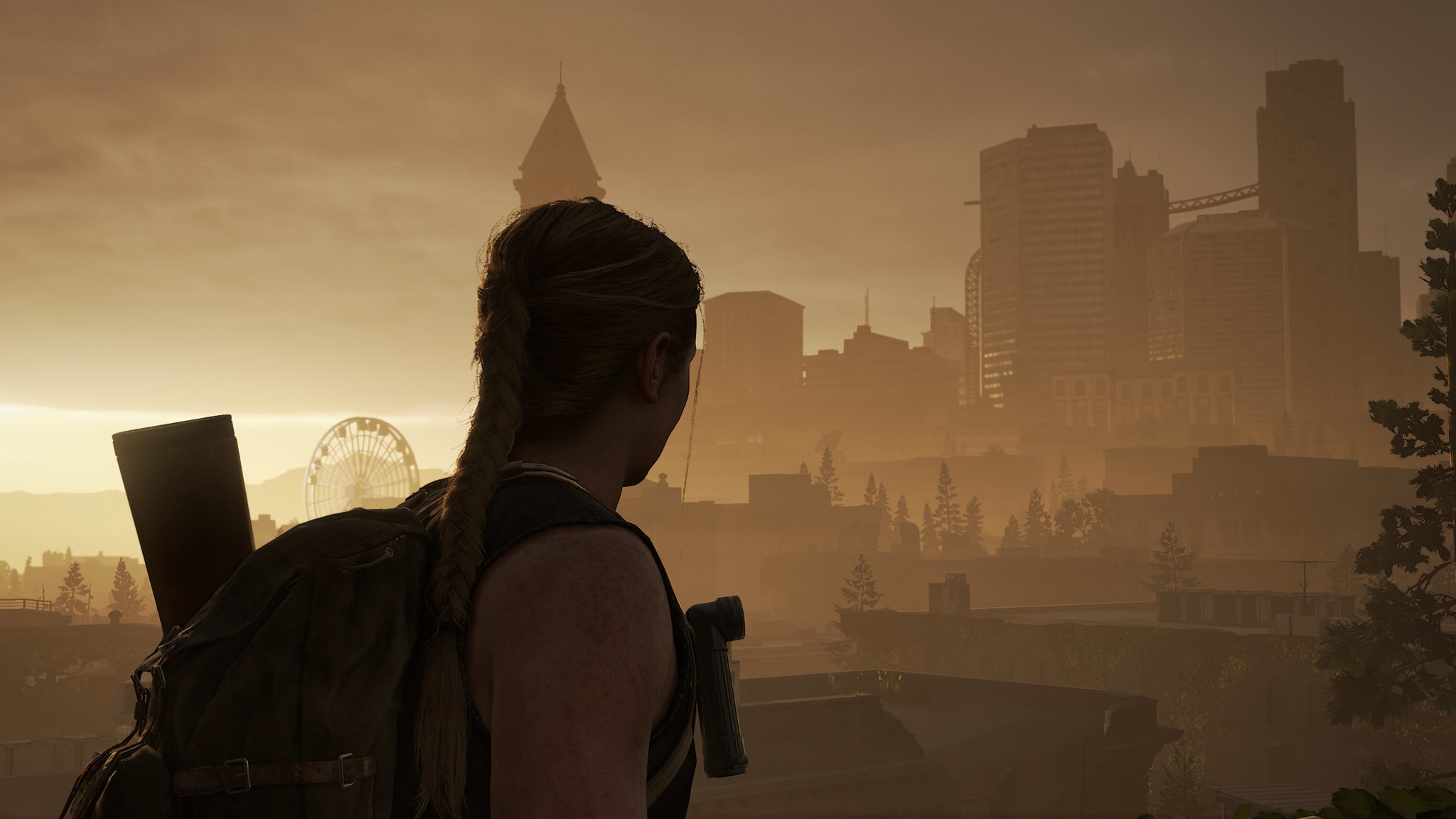In this screenshot from a video game, the camera is positioned in a third-person perspective, capturing the scene from behind the central character. The protagonist is a woman with light skin and blonde hair tied back in a ponytail, though her features are somewhat obscured by the backlighting casting her in shadow. She is dressed in a sleeveless shirt and carries a backpack. Attached to the front of her backpack is a flashlight, and just behind her, the stock of a rifle is visible, hinting at potential danger or adventure. The woman faces a distant city skyline dominated by tall buildings and skyscrapers, suggesting an urban setting. To her left, near the horizon, a Ferris wheel rises, adding a whimsical contrast to the otherwise stark scene.